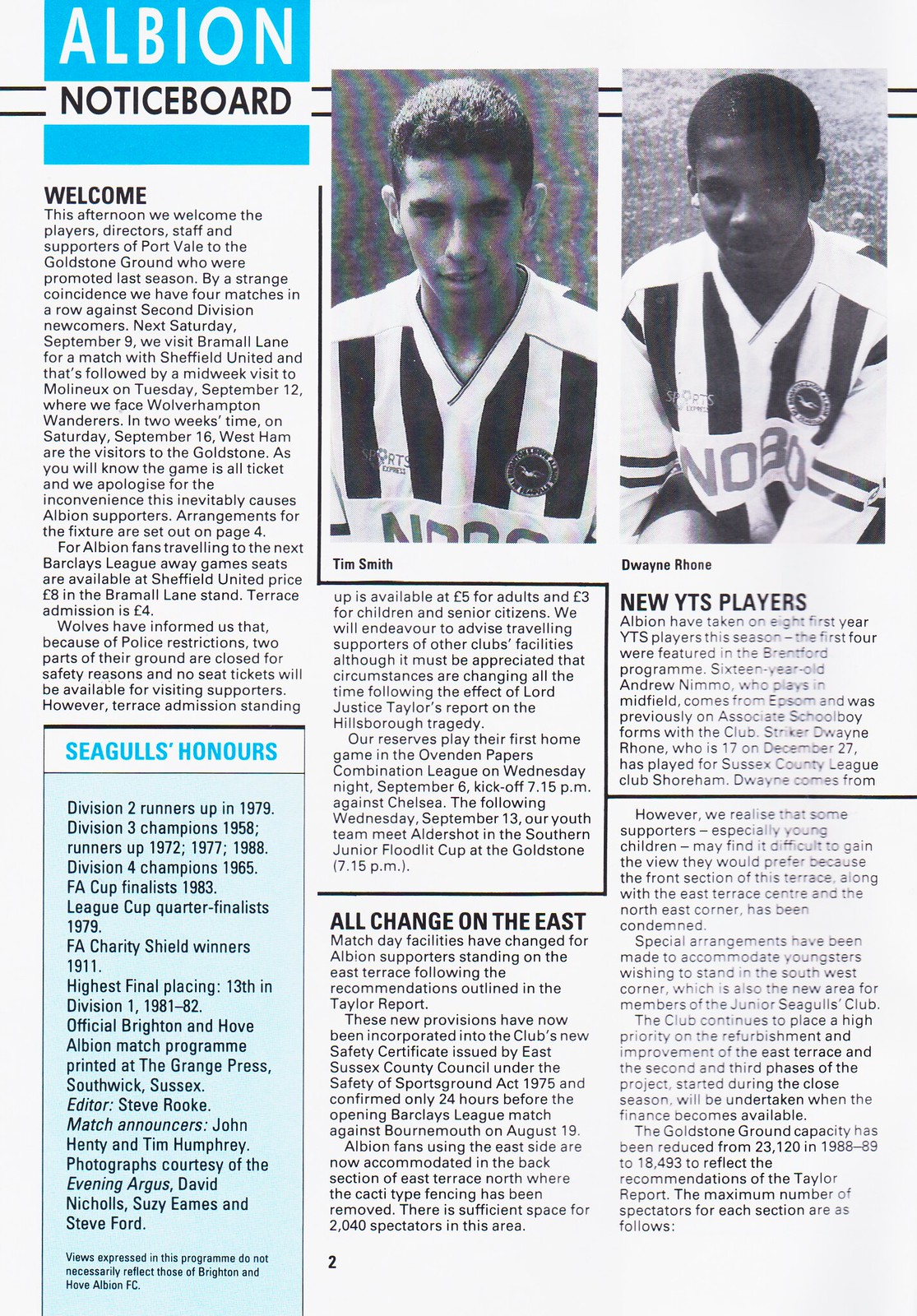The image depicts a detailed page from a soccer magazine styled as a noticeboard. Dominating the top of the page is a blue box with “Albion” inscribed in white font, and beneath it, in black font, is the word “Noticeboard.” The page is mainly divided into three columns filled with black text, including headings like "Welcome," "All Change on the East," and "New YTS Players." Towards the top right-hand side are two black and white photographs of soccer players. The player on the left is Tim Smith, and the player on the right is Dwayne Roan; both are identified below their respective images. Dwayne Roan is described as a black male, and Tim Smith also has darker skin. They are both wearing black and white striped jerseys. In the bottom-left corner of the page, there's a section titled “Seagulls Honors” in blue font, with additional black text underneath. Nearby, there is a small black number “2” indicating the page number. The page seems to welcome the players, directors, staff, and supporters of Port Vale to the Gladstone ground, reflecting on their recent promotions and upcoming matches against South Division newcomers.